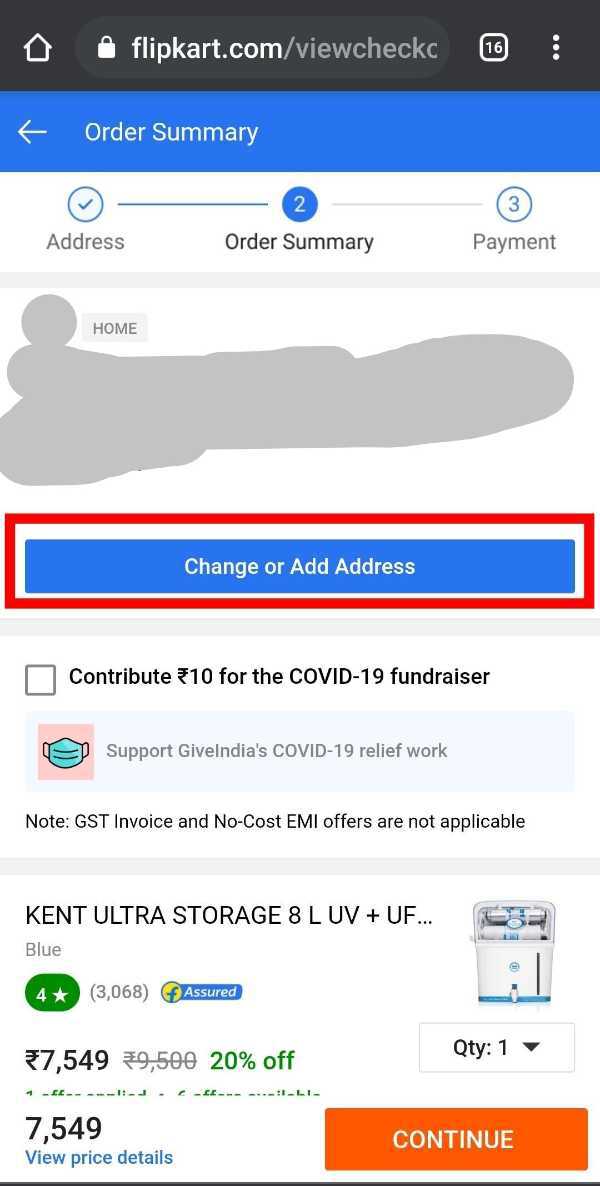The image features a structured user interface of what appears to be an online shopping website, displayed in meticulous detail:

At the top left corner, there is a black header featuring a simplistic white outline of a house, representing the home icon. Adjacent to it, the URL bar is highlighted, designed in an elongated oval shape with a dark gray background. On the left side of this bar, a white lock icon signifies a secure connection. The URL is prominently displayed in bold white text, reading "FLIPKART.COM/viewcheck," though part of the URL extends beyond visibility. To the far right of the URL bar, a small rounded square with "16" in white indicates the number of open tabs, followed by three vertical white dots symbolizing a dropdown menu.

Below the black header, a blue header features a left-pointing white arrow alongside the text "Order Summary" in white. Directly underneath, a white strip displays a circular blue outline icon with a blue checkmark inside, captioned "Address" in gray text. A blue line follows this, leading to another circular icon, this one filled with blue and showing a white number "2," labeled "Order Summary" in black beneath it. A light gray line separates this section from another circular icon bordered in blue, containing a blue number "3," under which the word "Payment" appears in gray.

Another minor gray line segment provides additional separation, followed by a small rectangular gray icon labeled "HOME" in dark gray, uppercase lettering. Part of the area is obscured by a light gray smudge, possibly indicating sensitive information or intentional redaction.

This detailed description captures the layout and elements meticulously, reflecting a well-organized online shopping navigation interface.